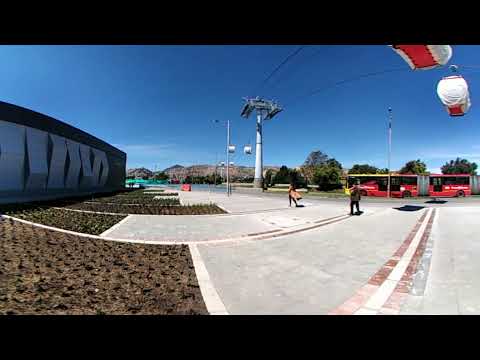The image features a busy scene near a large concrete building with graffiti on its far left side. The foreground is a gray parking lot with two people walking away from the camera, and the middle ground is dominated by a large red and yellow articulated bus traveling down a street. On the left of the image, there are rectangular planters filled with light brown soil and young green plants. Above the pedestrians, a gondola system can be seen, including white and red gondolas suspended from wires and a large support pole with a U-shaped beam. In the background, a mix of trees, additional buildings, and a distant dry mountain range under a clear blue sky can be observed, rounding out the scene with a touch of nature amidst the urban setting.